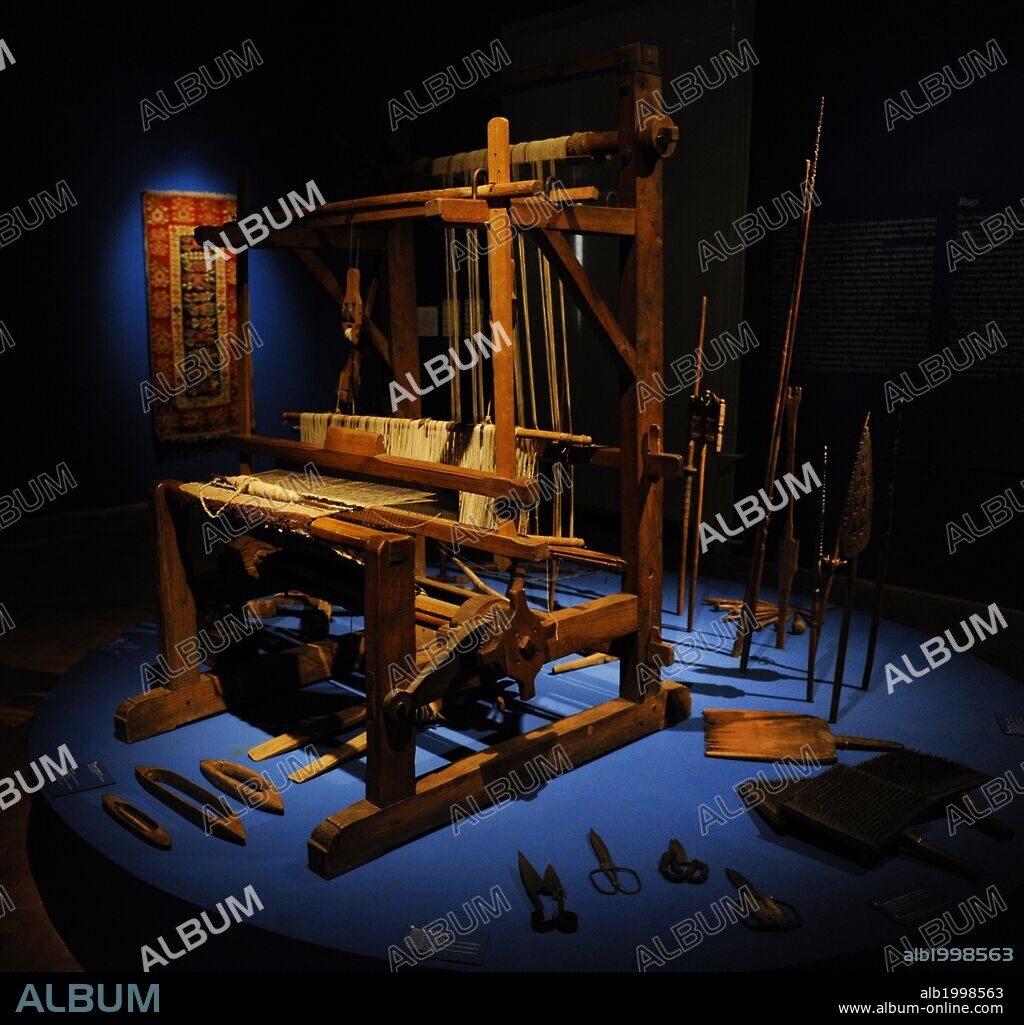The image features a vintage wooden loom prominently placed in the center of the frame, set against a dark, blackish-blue background with a spotlight highlighting its intricate details. The loom is equipped with thick, golden threads hanging down and appears ready for the weaving process. Surrounding the loom on the blue floor are various tools typically used in textile manufacturing, such as shears, iron scissors, and other wooden implements. To the left of the loom stands an elegant tapestry, partially hanging on the wall, adding a decorative touch to the scene. The image itself is watermarked repeatedly with the word "album" in various styles, including some instances with a white outline and others filled in white, while a black rectangle at the bottom of the image reads "album" in blue along with the text "ALB1998563" and a website URL, www.album-online.com.